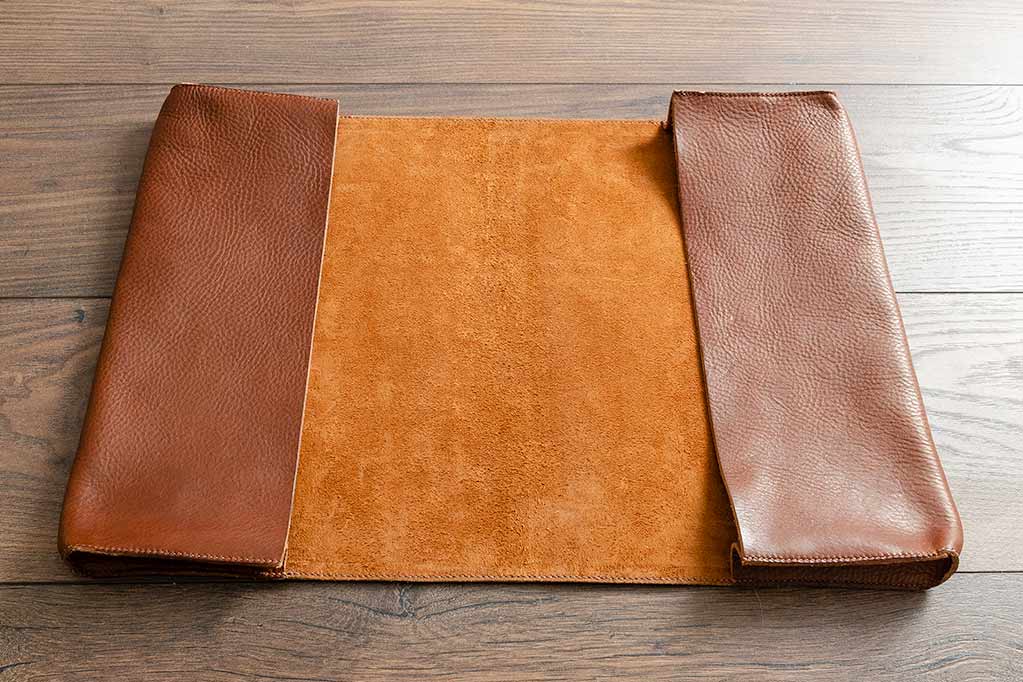The image features a rectangular leather cover or case, likely designed to hold a book, notebook, or similar item. The cover is made from brown leather and is laid open flat on a wooden surface, possibly a table or floor, which has a gray-brown hue and visible wood grain. The outer sides of the cover are a chocolate brown pebbled leather, while the interior, exposed in the center, is a lighter brown suede with an orange tint. Each side of the cover folds over to form a sleeve or pocket, where one could insert the covers of a book or other items. The stitching is visible around the edges, indicating a handmade quality. The leather displays highlights, particularly on the right side due to light coming from the upper right. The cover’s edges are rounded, and it has a rustic, traditional feel, evocative of a cowboy or ranch aesthetic. The entire object is devoid of any text, insignia, or fastenings like buttons or straps.